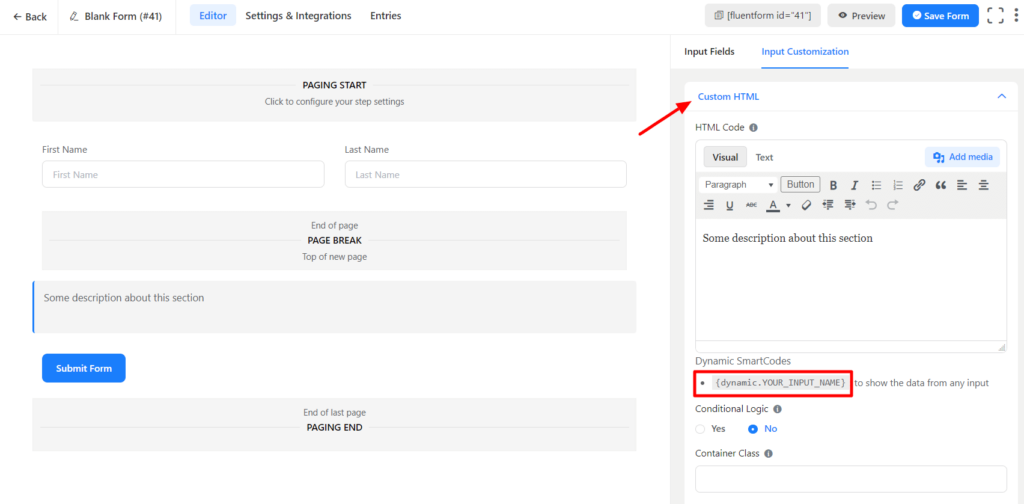**Screenshot of Smart HTML Coding Interface**

The image depicts a [software/interface] screenshot of an HTML coding editor designed for creating and customizing smart forms. The background is predominantly white, giving it a clean and structured appearance.

- **Header Section:**
  - At the top left, there is a black directional arrow pointing to the left accompanied by the text "Back" in black, a pencil icon, and the label "(41)" in parentheses.
  - A small gray rectangle with blue text labeled "Editor" comes next, followed by black text reading "Settings and Integrations" and "Entries".
  - On the right, a gray rectangle displays "Fluent Form ID = 41", adjacent to a smaller gray rectangular button with an eye icon and the word "Preview" in black text. Beside it is a prominent blue button titled "Save Form" in white text.

- **Main Content Area:**
  - A light gray rectangular banner states "Paging Start" in black text, followed by the instruction "Click to configure your step settings."
  - Below this banner are two side-by-side input fields labeled "First Name" and "Last Name."
  - Another gray rectangle, centrally positioned, reads "End of Page," followed by text indicating a "Page Break" and "Top of New Page."
  - The far left side has a blue vertical line running along the edge.

- **Section Descriptions:**
  - Below these input fields is an additional gray rectangle with the description "Some description about this section."
  - A blue button with white text at the bottom reads "Submit Form."

- **End Section:**
  - At the very bottom, another gray rectangle states "End of Last Page," with "Paging End" beneath it.

- **Customizations and Settings:**
  - To the right side of the screenshot, there is a segment with various input fields and settings.
  - Blue text labeled "Input Customization" is underlined, indicating a clickable link. Below it, "Custom HTML" is highlighted with a red arrow pointing diagonally upward to the right.
  - Next to it, "HTML Code" is noted in black text, followed by options for "Visual" and "Text" with an "Add Media" button to the right.
  - Another section at the bottom explains "Dynamic Smart Codes," outlined in a red rectangle with the description "to show the data from any input."
  - Below this, "Conditional Logic" is mentioned with a "Yes" or "No" option, with "No" being checked.

- **Additional Input Fields:**
  - The final part highlights a "Container Class" with a blank rectangle below for user input.

This descriptive caption thoroughly outlines the various sections, buttons, and functionalities presented in the screenshot of the HTML coding and form configuration interface.